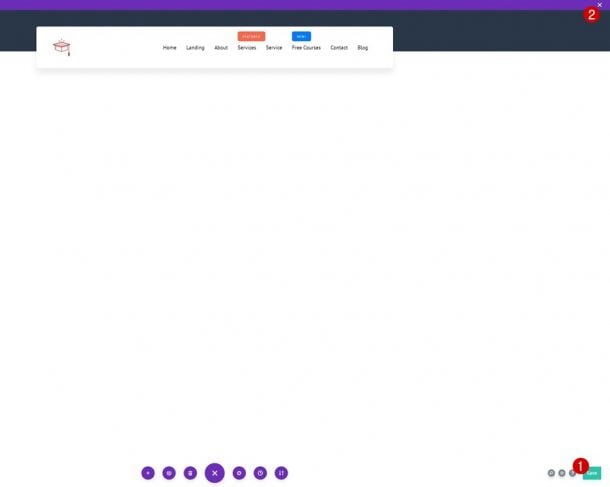The image depicts a mostly blank webpage with a predominantly white background. At the very top, there's a small purple navigation bar with a larger dark grey bar situated beneath it. In the upper right corner, there's a red dot displaying the number '2' in white font accompanied by a small 'X'. Inside the dark grey bar, a red graduation cap icon is visible within a banner. The bar also contains several tiny, unreadable category labels, except for a few visible words including 'Home', 'Learning', 'About', 'Services', and 'Science'. There is an orange bar above the 'Sciences' label and a blue bar above another label. The central portion of the page remains almost entirely blank. At the bottom, a series of purple circles with various icons are displayed, with the central and larger circle featuring an 'X' icon. In the bottom right corner, three brown circles are visible nearer a red circle labeled with the number '1' and a small, illegible green box. The overall impression is one of an incomplete or minimally populated webpage, potentially a tutorial, given its sparse content.